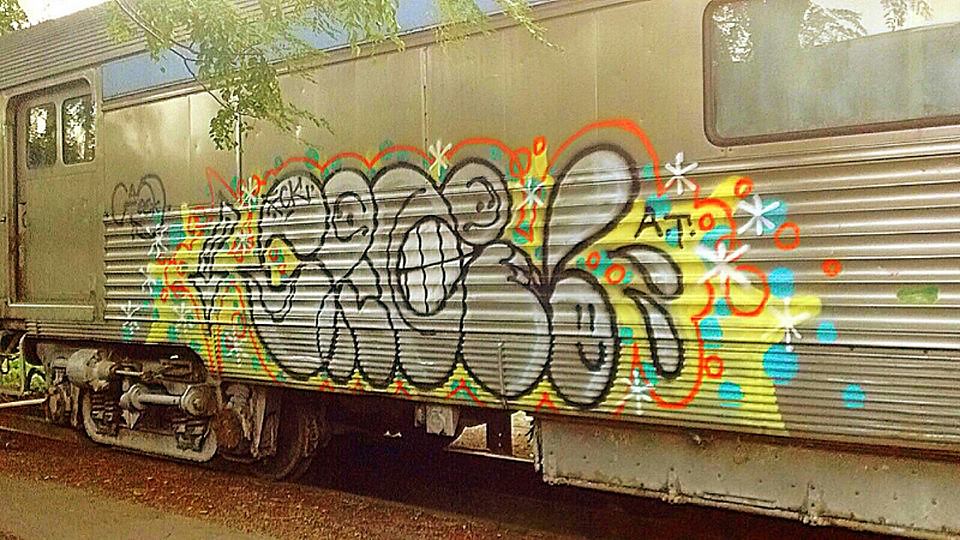The image shows an outdoor scene dominated by a large, horizontally-oriented, rectangular silver train car. Positioned on a railway track amidst lush greenery, the upper left corner of the photo reveals the sky and tops of green trees, with leaves gently resting on the structure. The train car, seemingly abandoned or out of service for a long period, is covered in dirt, grime, and even spots of moss, emphasizing its neglected state.

On the left side of the train car, there's a doorway featuring two small windows. To the right, another larger window is visible near the upper right corner. A blue band runs along the top of the car, adding a touch of color to the otherwise metallic surface.

The right side of the train car is extensively covered in vibrant graffiti. Various colors like yellow, gray, black, white, blue, green, and orange are splayed across the surface, creating a chaotic yet intriguing visual display. The graffiti includes gray circular faces, white star-like shapes, and scattered splotches of color. In the center of the graffiti is a depiction resembling cartoon teeth. This colorful and abstract art starkly contrasts with the dull and worn exterior of the train car.

The scene is illuminated by sunlight, which reflects off the windows and metallic surface of the train, adding a natural sheen to the otherwise gritty and aged appearance of the structure.